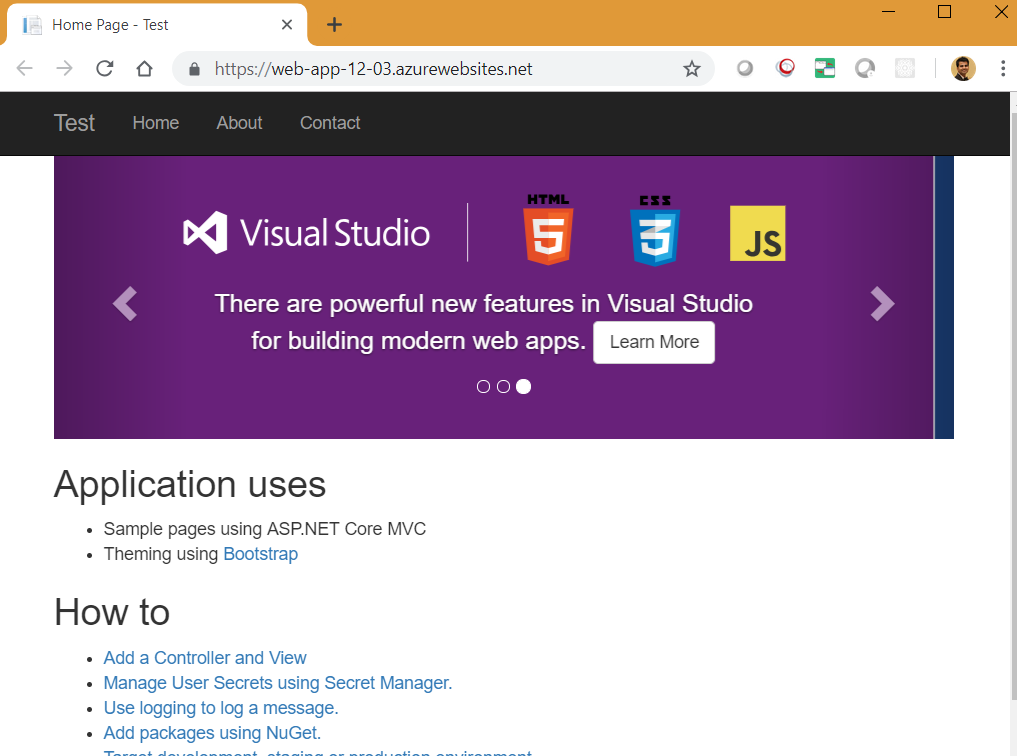**Detailed Caption for Image:**

This is a screenshot of a test home page, hosted on a secure HTTPS connection. The web address is displayed as "web-app-app-12-03.azurewebsites.net". To the right of the web address, there are a few icons including a star and others that are not easily recognizable, followed by a profile picture. Below the web address bar, there is a dark grey menu bar with navigation options labeled as "Test", "Home", "About", and "Contact", with "Test" being the largest and most prominent text.

The main content begins with a large purple field that contains a vertical blue bar on the right. On this field, the Visual Studio icon, which consists of two opposing triangles, is prominently displayed on the left. Adjacent to this, there are logos for HTML5, CSS3, and JavaScript in their respective colors.

A white button with the text "Learn More" invites users to explore powerful new features in Visual Studio for building modern web applications. Below this, a segment titled "Application Uses" showcases sample pages created using ASP.NET Core MVC and Bootstrap for theming.

In the subsequent "How-To" section, various instructional links are provided in blue text with bullet points. The options listed include "Add a Controller and View," "Manage User Secrets with Secret Manager," "Use Logging to Log a Messenger," and "Add Packages Using Gnet." The rest of the content is cut off in the screenshot.

This comprehensive layout highlights both the navigational structure and the functional capabilities offered on the home page test for a web application hosted on Azure.